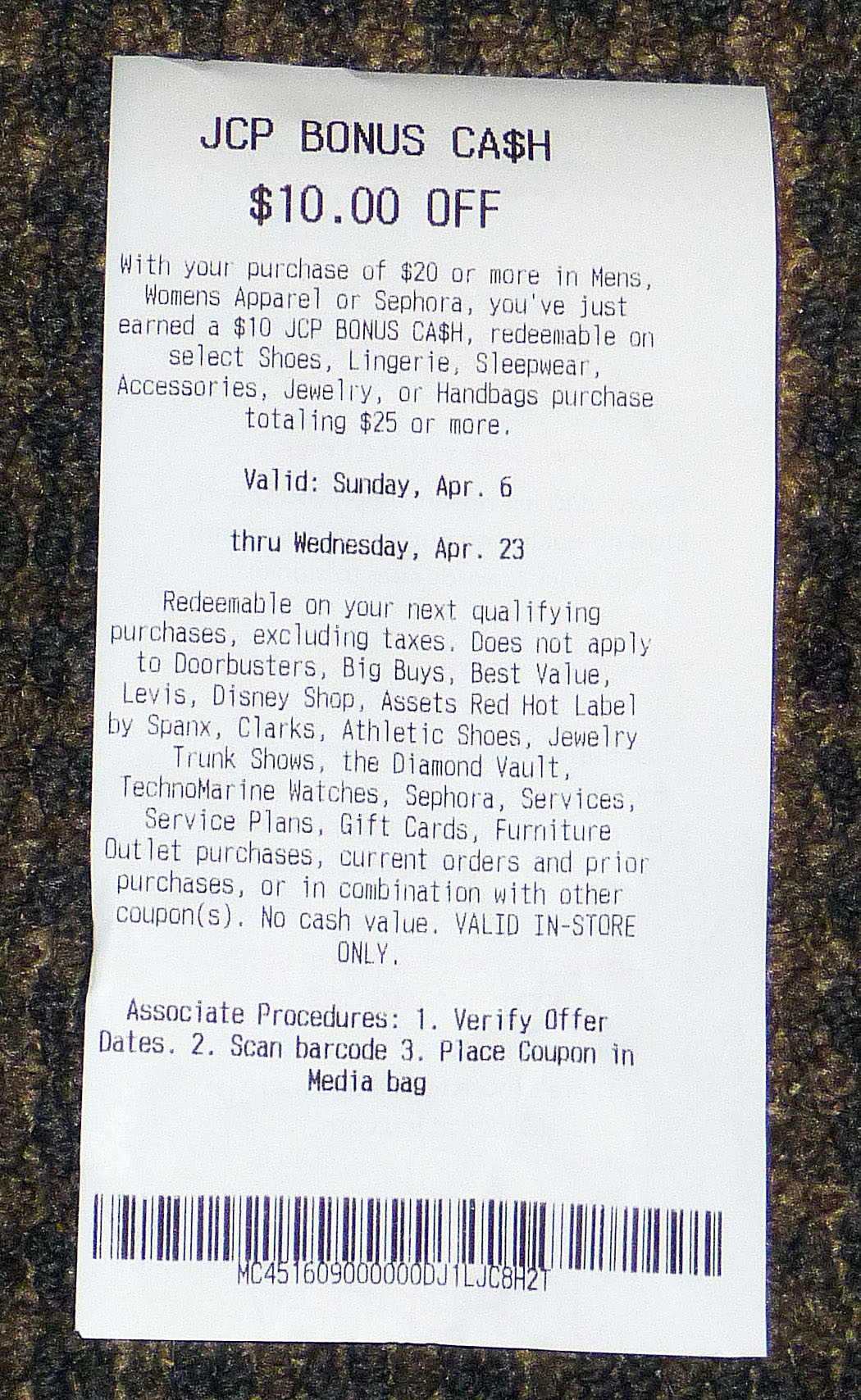In this photograph, we see a JCPenney receipt prominently displayed against a textured, wooly carpet background in brown with black gradient hues. The receipt itself is white with black text, clearly showing details of a promotional offer.

At the top, the receipt highlights a $10.00 JCP Bonus Cash award, which is applicable with a purchase of $20 or more on men's and women's apparel or items from Sephora. The text outlines that the earned $10 bonus cash can be redeemed on select shoes, lingerie, sleepwear, accessories, jewelry, or handbags totaling $25 or more. The valid period for this offer is from Sunday, April 6th through Wednesday, April 23rd.

Several exclusions are noted on the receipt, stating that the bonus cash does not apply to door busters, big buys, best value items, Levi's, the Disney shop, assets by Spanx, Clarks footwear, athletic shoes, jewelry trunk shows, diamond vault items, Technomarine watches, Sephora products, services or service plans, gift cards, furniture outlet purchases, and both current and prior orders or purchases in combination with another coupon.

The bottom of the receipt lists specific associate procedures for handling the coupon: Verify the offer dates, scan the barcode, and then place the coupon in the media bag. This detailed accounting ensures clarity in the redemption process and assists in maintaining store procedures.